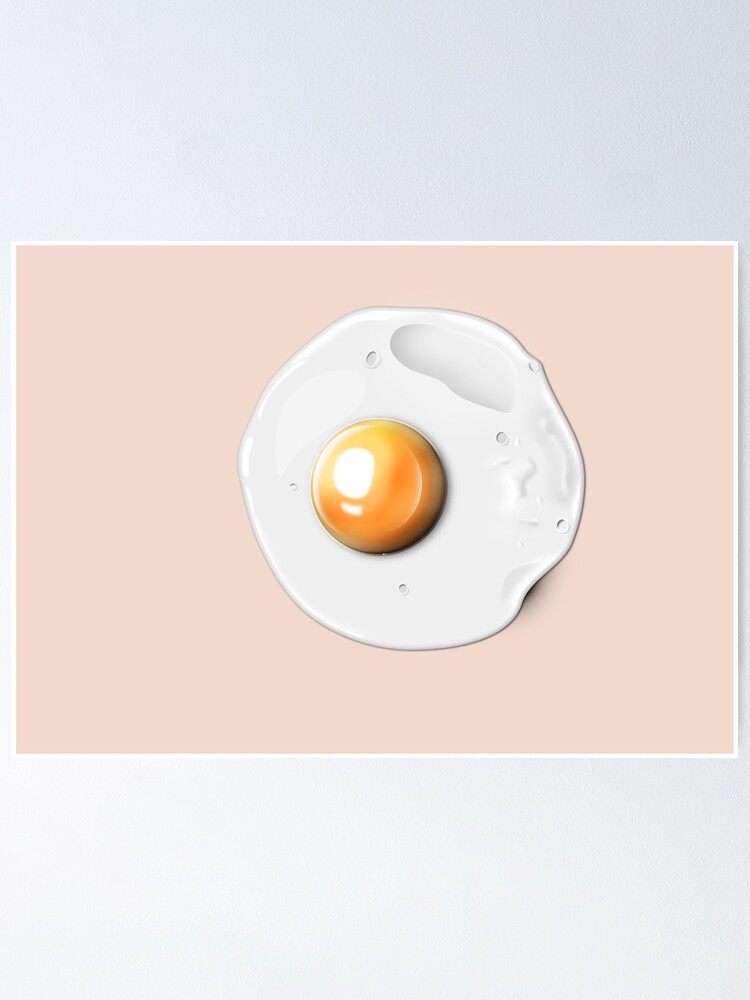The image depicts a sunny side up egg with a perfectly circular, golden-yellow yolk that appears intact and slightly runny, surrounded by a solidified white egg white. The egg itself has a somewhat cartoonish, drawn appearance, further emphasized by the light reflections and grayish craters on the egg white. This artistic rendering of the egg is set against a pale pink triangle backdrop, which is mounted on a light grayish-white background, giving the entire scene a clean, minimalist look. The detailed design and layered background make it a visually appealing and whimsical representation of a simple fried egg.